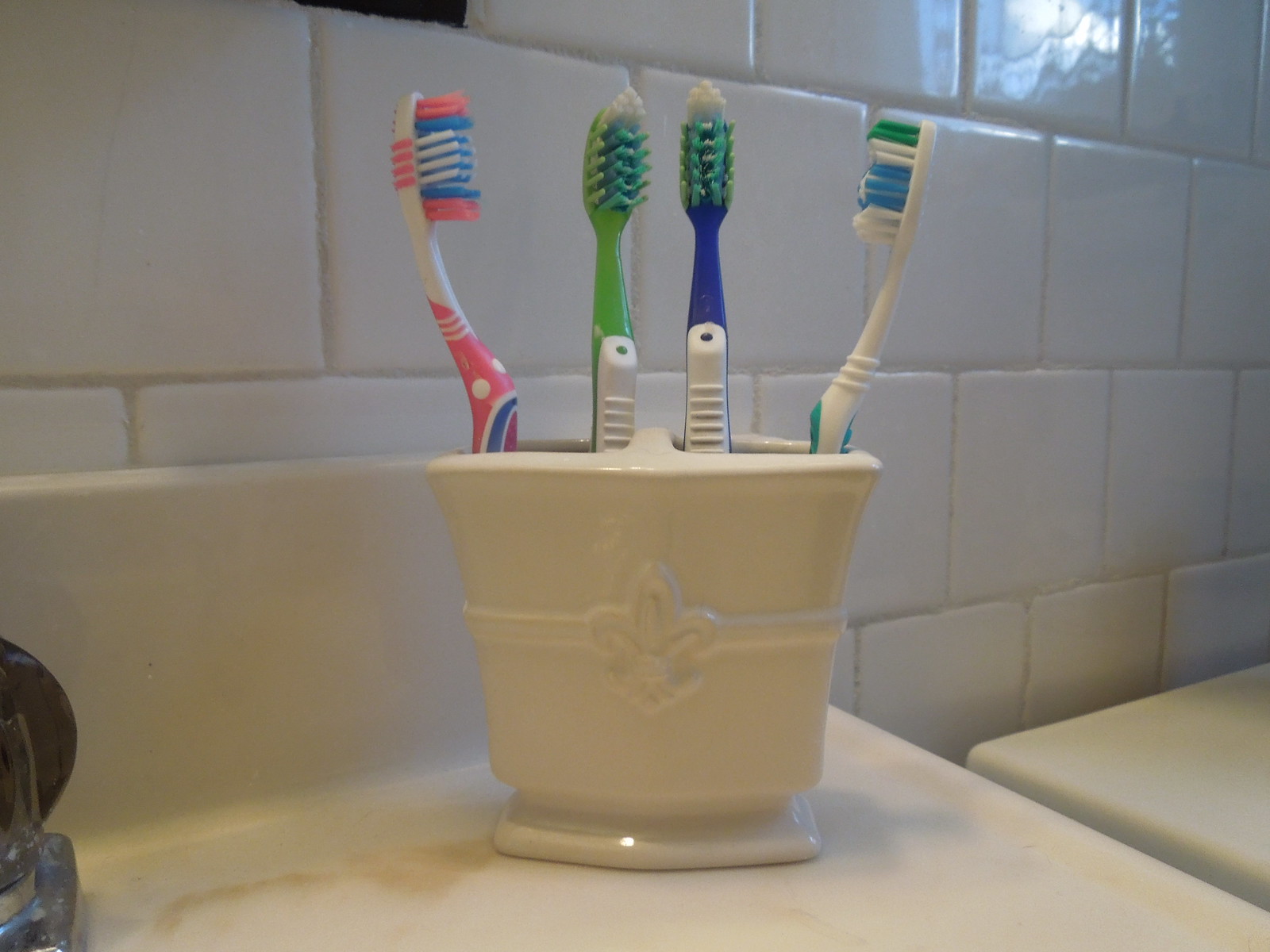This photograph features a detailed close-up of a white porcelain toothbrush holder adorned with a central fleur-de-lis decorative embossing. The holder has a sleek design with a wide base that narrows in the middle before flaring out at the top. Placed on a white marble surface in a bathroom with a shiny white tiled wall arranged in a brick pattern, the toothbrush holder organizes four colorful toothbrushes distinctively arranged in a semicircle with their bristles facing inward.

The toothbrushes include: the leftmost one with a pink shaft accented by blue and white decorations and bristles in pink, blue, and white; the second with a green and white shaft featuring bristles in green, blue, and white; the third with a blue and white shaft and matching bristles in blue, green, and white; and the rightmost toothbrush with a predominantly white shaft with blue highlights and bristles in blue, green, and white. 

None of the toothbrush heads are touching, maintaining a neat and orderly appearance. There is a glimpse of a stainless steel tap at the bottom left of the frame, and a subtle reflection of light from a nearby window can be seen on the white tiles. The immaculate arrangement and the floral detail of the holder create an aesthetically pleasing and harmonious setup.